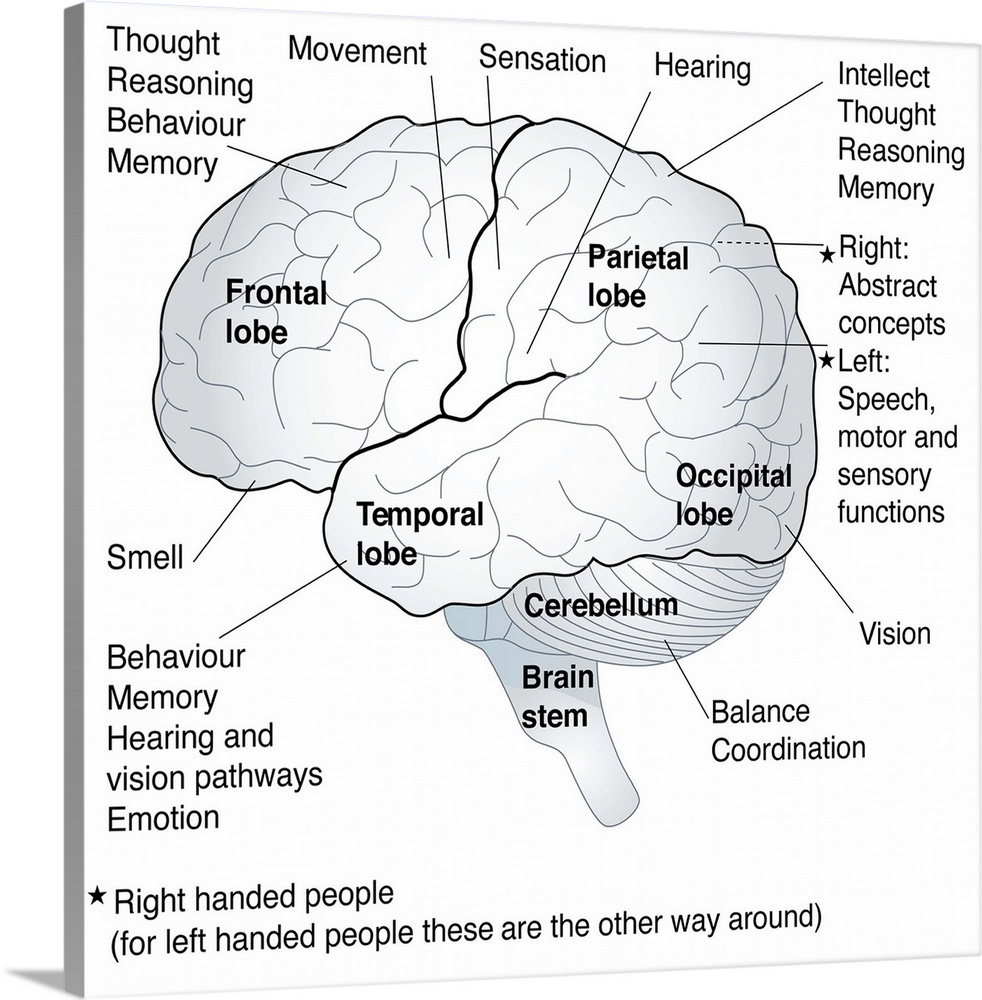This image is a detailed, black-and-white graphical representation of the human brain on a white background. The brain is colored gray with distinct black outlines and is sectioned into different lobes, each labeled with its specific functions. Arrows and word bubbles radiate from various parts of the brain, pointing to its roles and responsibilities. 

In the top left, the frontal lobe is indicated and associated with thought, reasoning, behavior, memory, movement, and smell. The parietal lobe, located on the right, is responsible for sensation and hearing. The occipital lobe, situated towards the left, is dedicated to vision. Below these, the cerebellum is highlighted for balance and coordination, and the brainstem is depicted too. The temporal lobe, noted for behavior, memory, hearing, vision pathways, and emotion, is also prominently featured.

Additional details include descriptors for intellectual thought, reasoning, memory, and abstract concepts, pointing towards respective areas. A special note highlighted with a star at the bottom left mentions right-handed people and how these functions may differ for left-handed individuals. The image is presented in a minimalist style, utilizing only black ink for labeling against a white canvas or paper background, emphasizing the brain's anatomical and functional divisions.